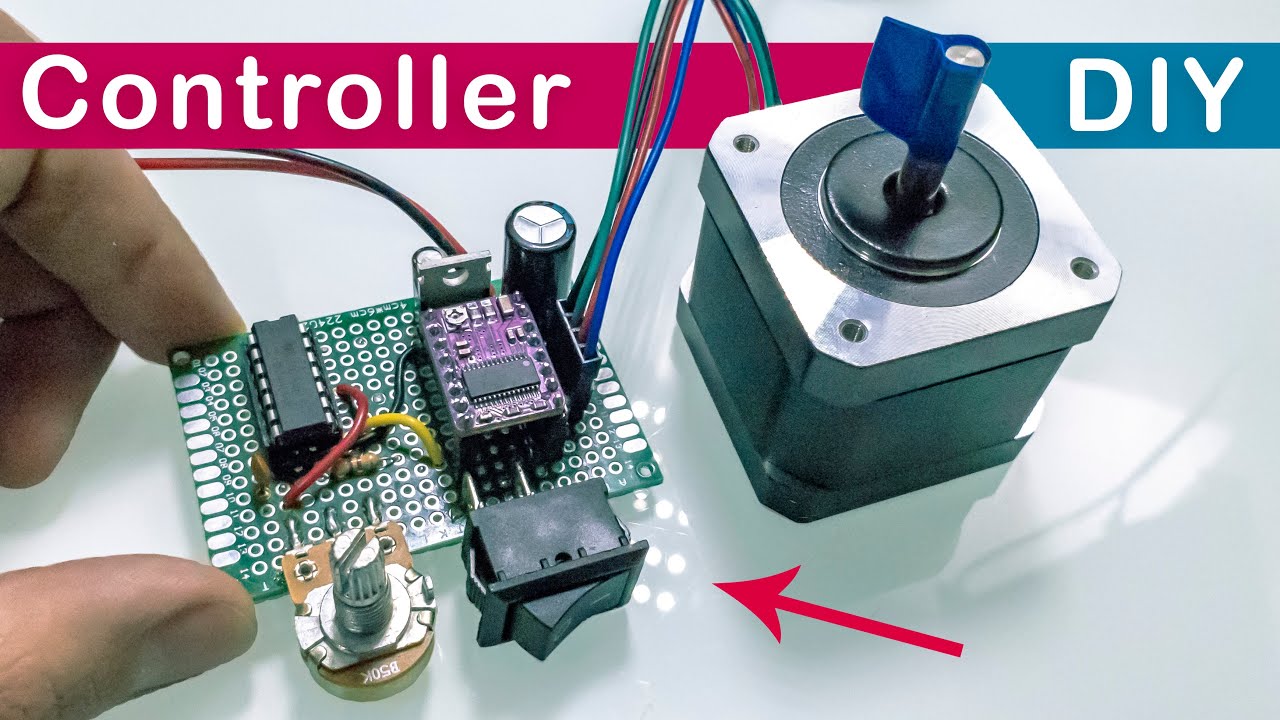The image depicts a detailed setup of a DIY electronic device. At the top, text reads "Controller" in white font on a red background to the left and "DIY" in white font on a blue background to the right. The background is a highly reflective white surface. The main focus is a square controller with a joystick at the top, covered in blue tape. This controller appears in the second third of the frame. There are three wires—red, green, and black—emerging from the controller and extending out of the image at the top.

Additionally, four wires—green, black, red, and blue—enter the frame and connect to a complex control panel adorned with various electronic components. This control panel includes switches and is mounted on a green circuit board, which the person's left hand is holding between their thumb and index finger. Also visible are three other wires—red, yellow, and black—attached to this circuit board. A red arrow points towards the green board, emphasizing it as part of the DIY setup. This image showcases a hands-on, intricate assembly of electronic components, suggesting a functional purpose, although its exact use is unknown.